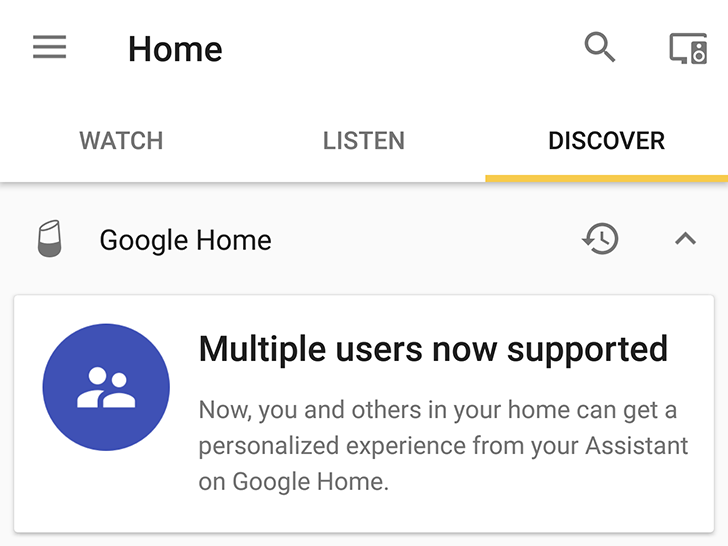The image is a screenshot of a Google Home notification displayed on a clean, white background. In the upper left corner, three horizontal gray lines represent a menu or more options. Next to it, the word "Home" is written in bold, black lettering. On the far right, a gray magnifying glass icon serves as the search function, accompanied by a gray computer screen with a speaker icon.

Just beneath these icons, there are three sections labeled "Watch," "Listen," and "Discover." The "Discover" section is in bold black font and underlined in yellow, indicating it is the currently active tab, whereas "Watch" and "Listen" are both in gray.

Below this, there is a small gray Google Home icon with a dark base and a lighter top, accompanied by the text "Google Home" in black font. On the right-hand side of this text, an icon resembling a refresh symbol with an upward-pointing arrow is displayed.

The main content is set inside a white box, featuring a blue circular icon with two figures, alongside the message: "Multiple Users Now Supported. Now you and others in your home can get a personalized experience from your assistants on Google Home."